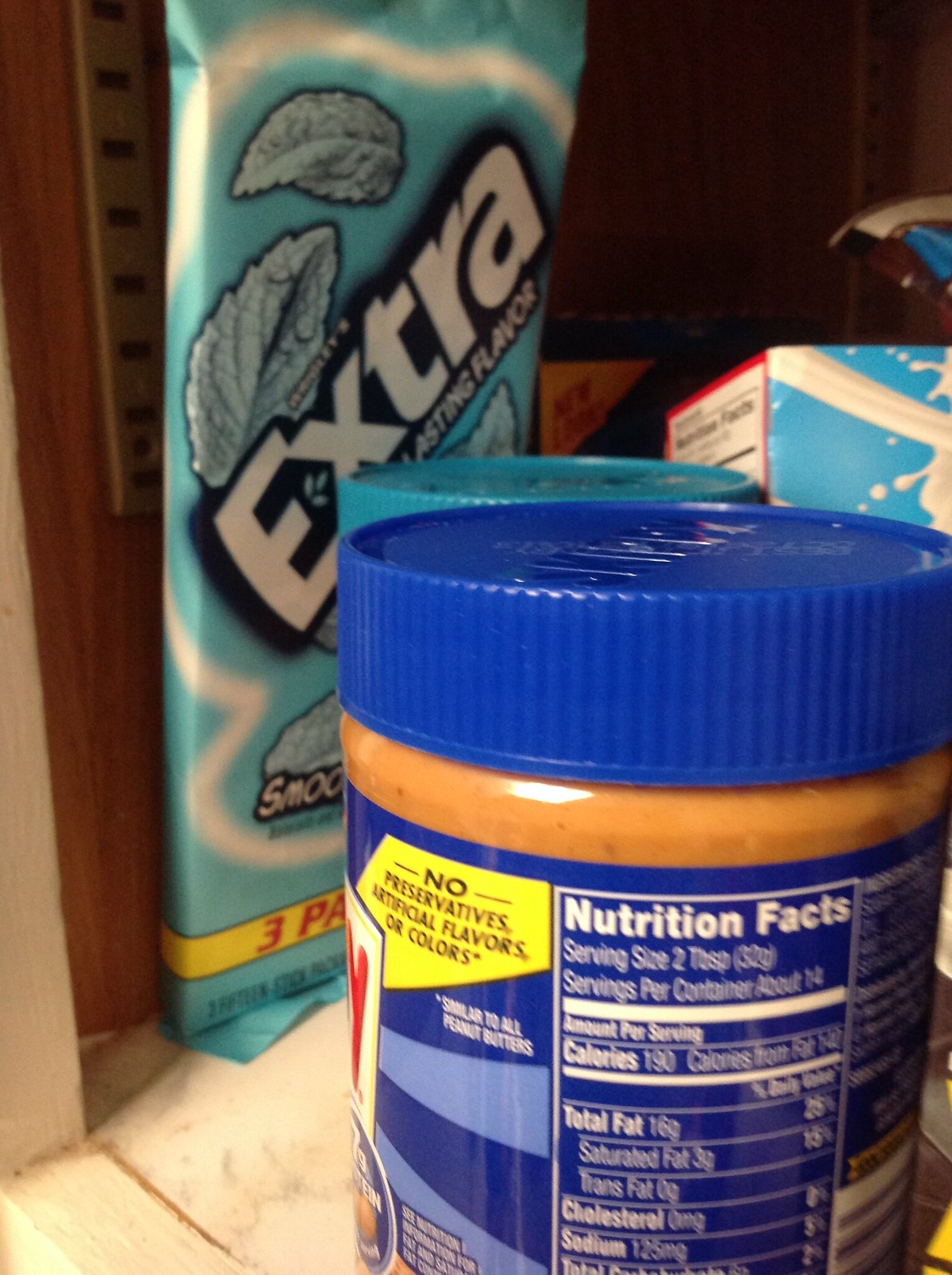This photograph captures the interior of a wooden cabinet, revealing its bottom and left wooden panels. A metal shelving arm is affixed along the left side, extending upwards. The cabinet's interior is a rich brown wood, adding a warm, rustic hue to the scene. 

Inside, a prominently visible jar, likely of Skippy peanut butter, features a blue label with white font and a matching blue lid. Positioned behind it, another jar with a teal-colored lid peeks through. A scratch pad or cleaning pad leans against the left side of the shelving, suggesting practicality and regular use. Various other boxes and bags are scattered throughout the cabinet, though their contents remain indiscernible. The overall composition offers a glimpse into an everyday storage space, filled with commonplace household items.